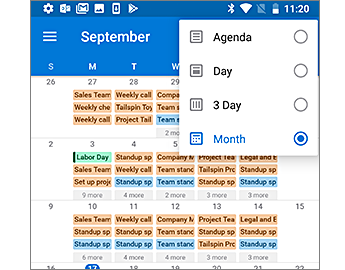This image is a cropped screenshot of the "Month" view tab in a calendar app. The top portion of the screenshot features a dark blue phone banner containing various icons. On the top left, several icons are visible including settings, Google Mail, a phone icon, and a small calendar icon. The top right displays the Bluetooth icon, signal strength, battery indicator, and the current time.

In the upper-right corner, there's a pop-up menu with bullet points (or radio buttons). To the left of this menu are options labeled "Agenda," "Day," "3 Day," and "Month," with "Month" being the selected view.

Beneath the phone banner is a lighter blue banner displaying the month "September." The days of the week are listed horizontally at the bottom of this banner. Following this are the dates for the last week of September: Sunday the 26th, Monday the 27th, Tuesday the 28th, and so on.

Specific dates in this calendar view are highlighted in different colors: some dates are marked in orange and others in blue, indicating scheduled events. Notably, Labor Day is highlighted in light green, drawing special attention.